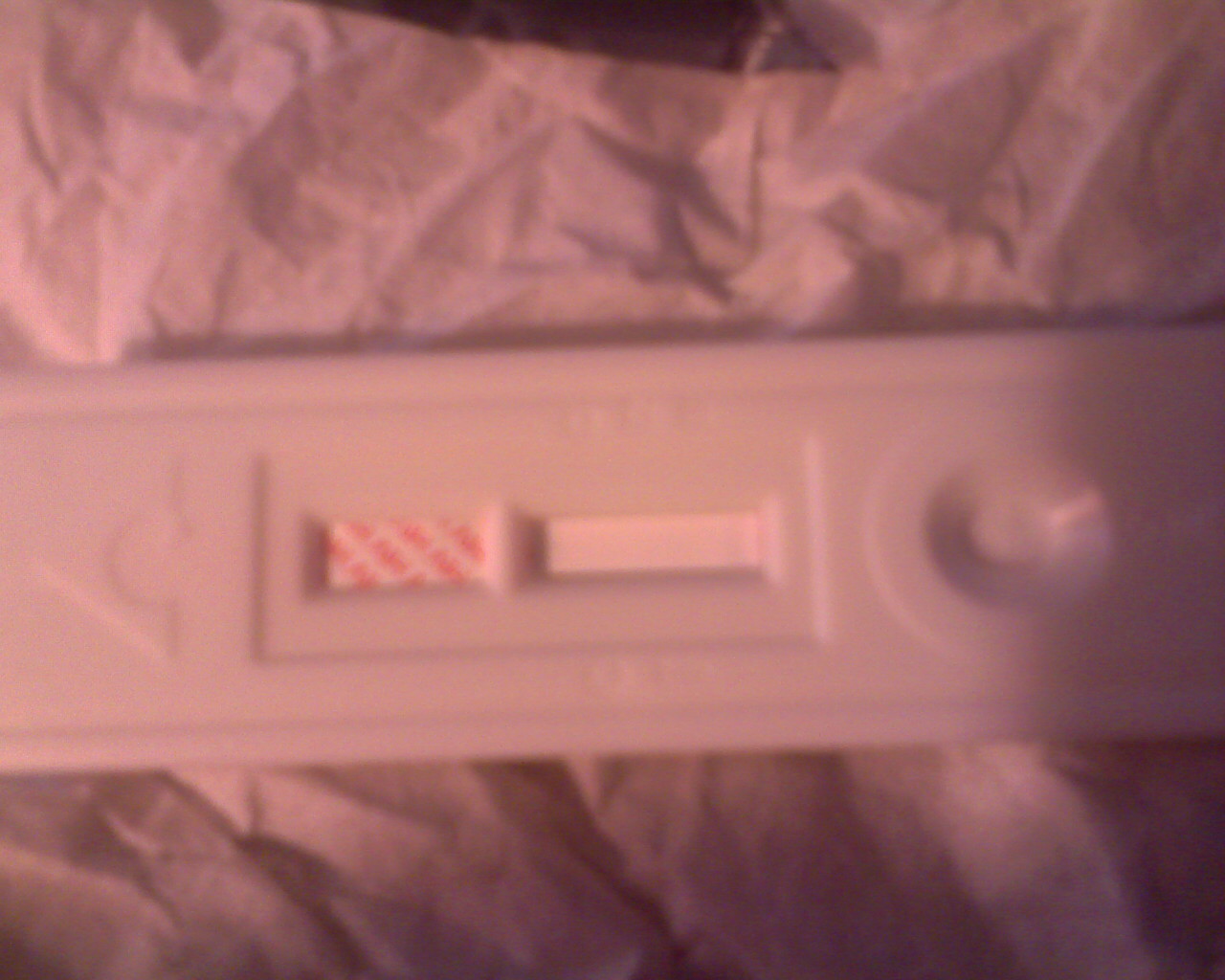A highly zoomed-in, somewhat blurry image depicting a test strip, which appears to be from either a pregnancy test or a COVID-19 test. The test strip is the main focus, though due to the blur, the specific details and results are unclear.